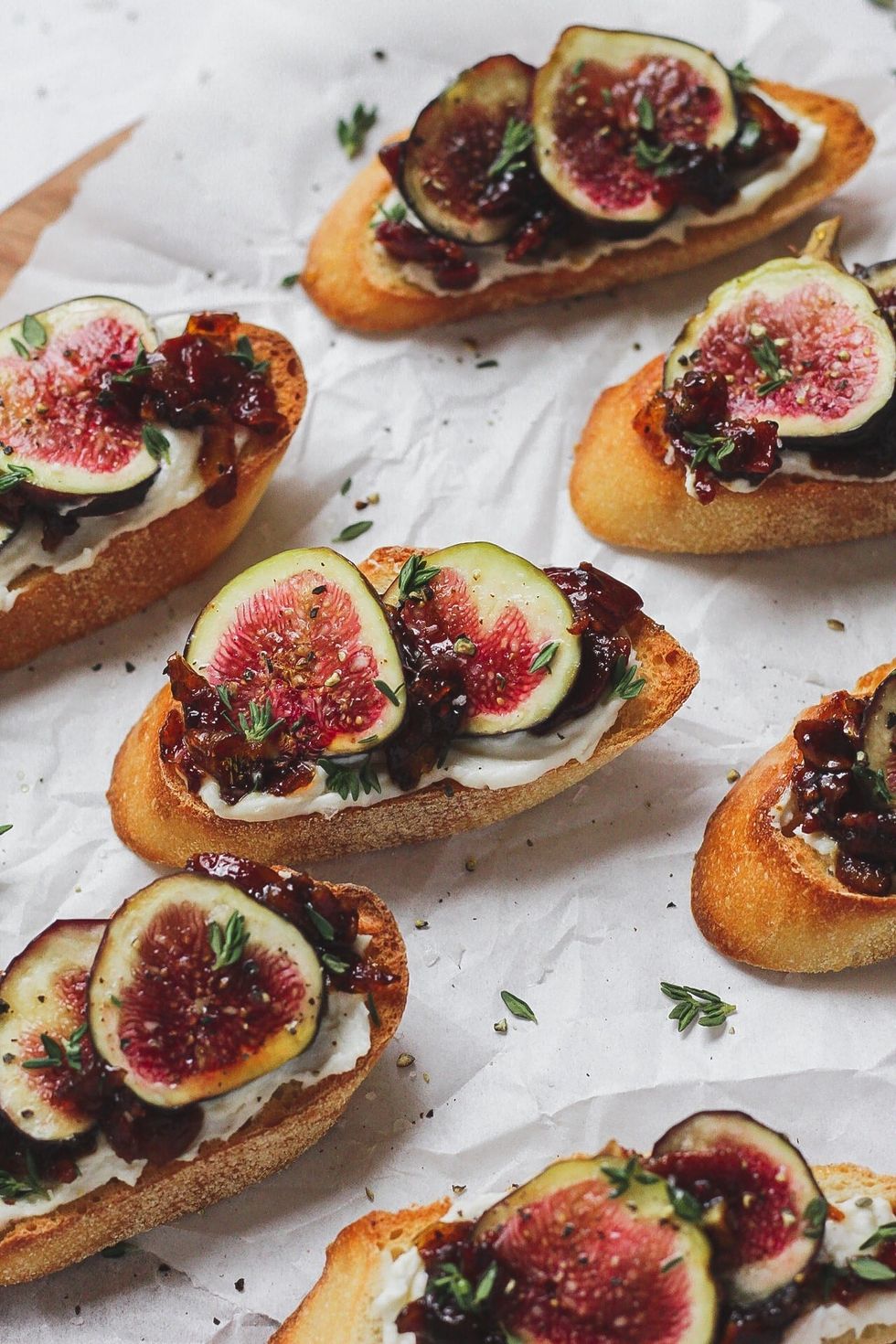The photograph captures a professionally staged, culinary image showcasing an array of elegantly prepared fig and goat cheese crostini appetizers. These crostini consist of lightly toasted slices of Italian bread, each adorned with a layer of creamy goat cheese. Atop the cheese sits a slice of fresh fig, showcasing its vibrant red pulp speckled with tiny black seeds and encased in a green outer skin. To enhance the flavor and presentation, the crostini are further embellished with drizzles of fig jam, honey, and a sprinkle of black pepper. Fresh thyme leaves and other tiny green seasonings are scattered artfully over the crostini and the surrounding parchment paper, suggesting a just-prepared and ready-to-serve state. The image is vertically rectangular, with a crisp white cloth background that amplifies the rich colors and textures of the meticulously arranged appetizers, creating an inviting, gourmet visual appeal.